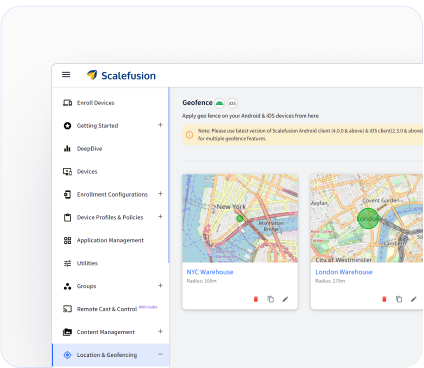**Descriptive Caption:**

A detailed screenshot of the Scale Fusion website interface is depicted. The website's name, "Scale Fusion," prominently appears in the upper left corner. Directly below, a vertical navigation column occupies the left third of the image, listing several options including Enroll Devices, Get Started, Deep Dive Devices, Enroll Configuration, Device Profiles and Policies, Application Management, Utilities Groups, Remote Casting Control, and Content Management.

To the right of this navigational column is the main content area featuring a section titled "Geofence." Within this section, there are two maps displayed side by side. The first map on the left illustrates a street map of lower Manhattan, labeled as "NYC Warehouse." The second map on the right shows a street map of central Westminster, labeled as "London Warehouse." Above these maps, an instructional text reads, "Apply Geofence on your Android and iOS device from here." Additionally, there is an unreadable pop-up notification window below the maps, suggesting some form of a user alert or update.

Overall, the interface seems to guide users on how to apply geofencing options to their devices, with various functionalities accessible through the left-hand menu and specific map locations provided as illustrative examples.